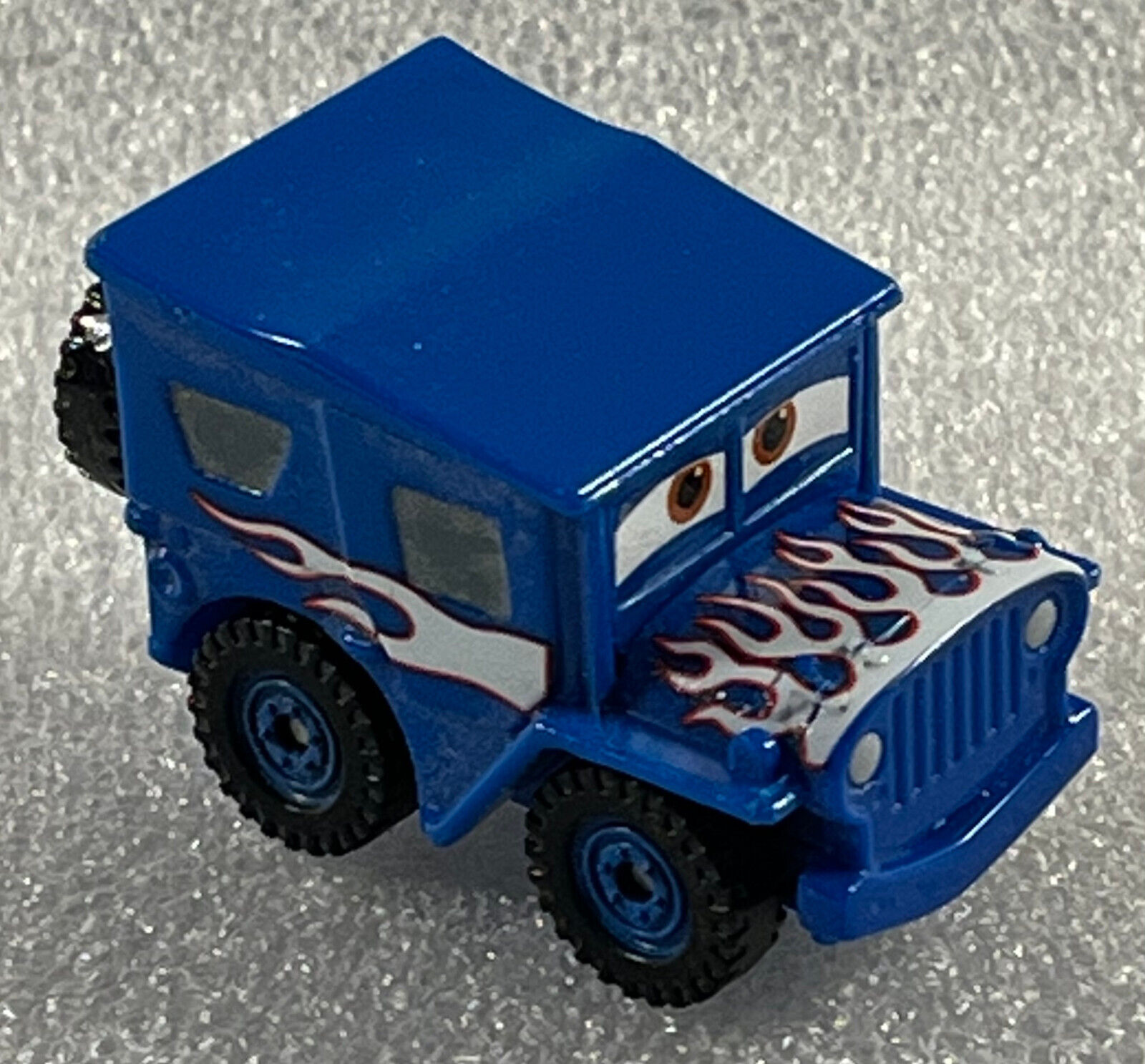This image showcases a small toy car, roughly 2 by 1 inches in size, resembling a character from the Disney-Pixar movie "Cars." The vehicle is styled as a dark blue Jeep with vivid white flames adorning the hood and sides. The front windshield features a pair of expressive, slightly cross-eyed brown eyes, characteristic of the anthropomorphized cars in the film. Equipped with large black tires and blue hubcaps, the toy also sports a blue grille, blue bumper, and a solid blue roof with two side windows. A spare tire is mounted on the back, enhancing its rugged appearance. The backdrop is a slightly blurry, white, and cream-colored carpet.